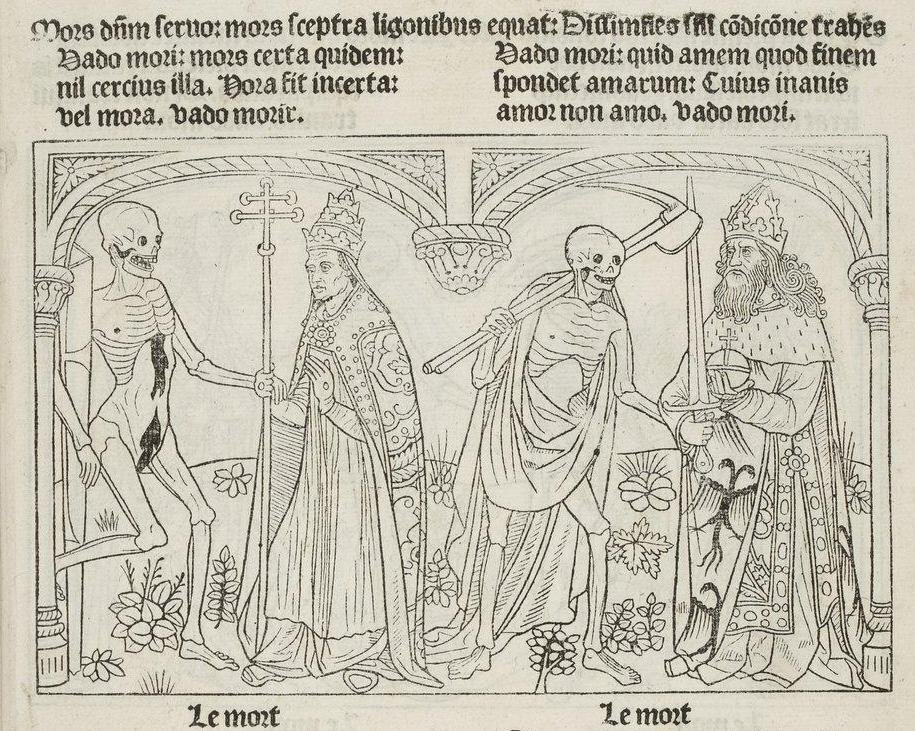The image depicts intricate line art illustrations on a beige parchment, reminiscent of medieval artistry, with a flat, pre-perspective style. Central to the scene are two pairs of figures: on the left, a religious figure, possibly a bishop or pope, adorned in ornate robes and headgear, holds a staff with an elaborate top. He faces a skeletal figure dressed in draped fabric and wielding a scythe, symbolizing death. On the right, another kingly or religious figure in a long coat and a crown-like headpiece clasps an orb and a sword. He confronts a second skeletal apparition, which is less draped and more menacing in form, extending a bony hand to grasp the staff.

The background features arches, columns, and a patterned field adorned with flowers and plants, contributing to the overall ornate composition. Above and below each pairing, blocks of text, possibly in Latin, frame the illustration, while the words "La Mort" (French for "death") are inscribed beneath each scene. This visually and contextually rich artwork encapsulates the inevitability of death confronting both nobility and the ecclesiastical elite.